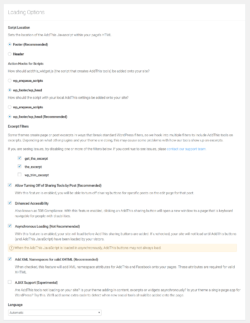This image depicts an exceptionally small, unreadable segment of a website, dominated by a gray background and a layout that primarily consists of dense textual information. The text varies in color, with some content in an extraordinarily light gray that's nearly indiscernible, while other parts stand out in bolder black fonts. The content is organized in a vertical bullet-point format along the side of the screen, with the bullets resembling check marks. 

Although the majority of the image features plain text, there are a few key details: one item includes a sentence highlighted in blue, presumably a clickable link for further information, and another is emphasized with a beige background. However, due to the minuscule size and the overall blur that intensifies with proximity, the specific details and purpose of the text remain completely illegible, even with readers. The entire visual suggests an overload of written information rendered ineffective by its diminished scale and clarity.